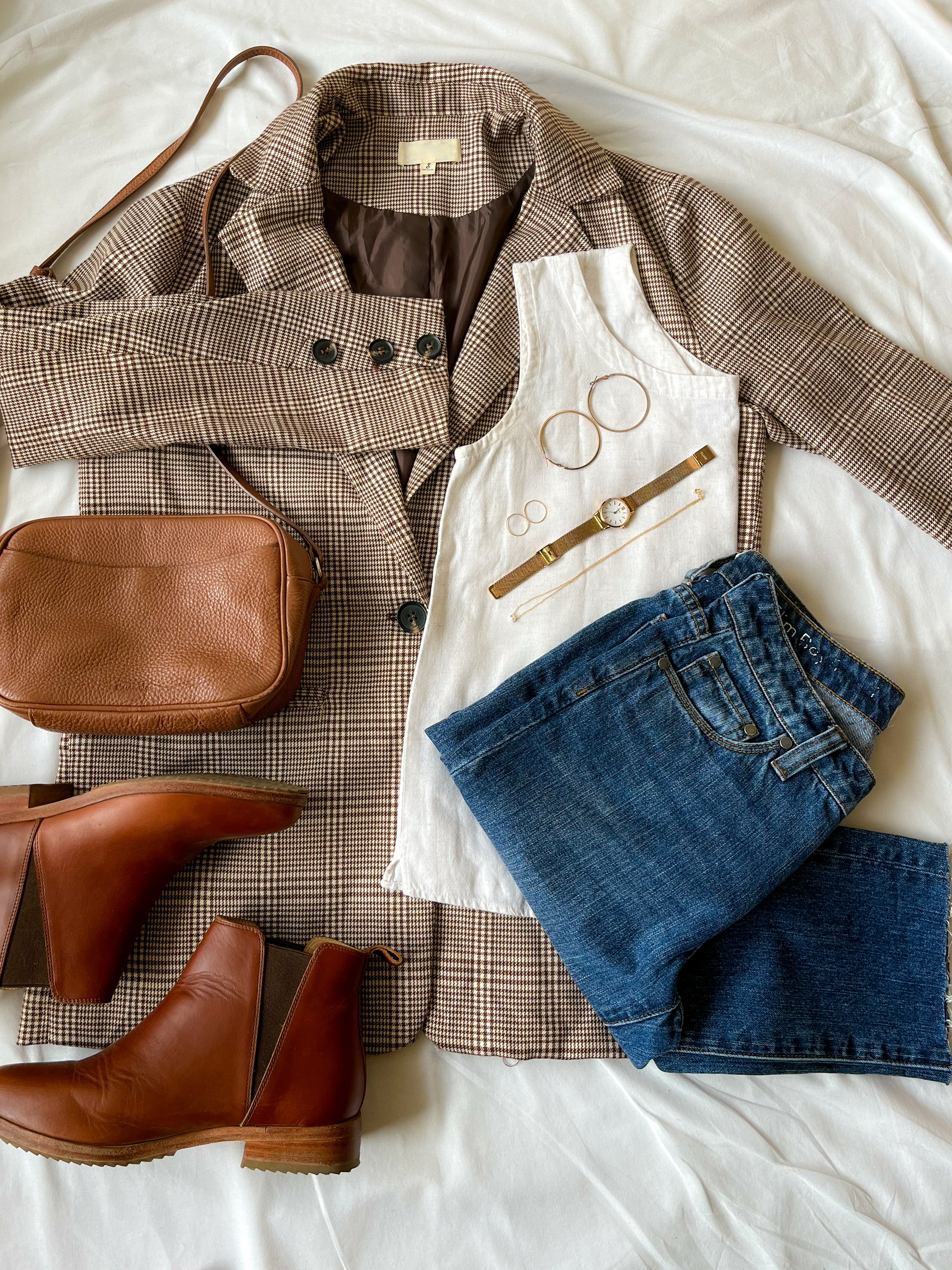This image, reminiscent of a stylish fashion magazine or a Pinterest layout, showcases a women's outfit meticulously arranged against a white fabric backdrop, likely a blanket or sheet. The focal point is a plaid brown blazer adorned with black buttons, paired seamlessly with a white camisole underneath. A pair of blue jeans is neatly folded next to the blazer, adding a touch of casual elegance. Complementing the outfit are sleek, ankle-high leather boots and a small brown leather shoulder bag, perfect for a chic, cohesive look. Gold accessories, including large hoop earrings, a wristwatch, two rings, and a bracelet, enhance the ensemble’s elegance. This thoughtfully curated outfit is ideal for occasions ranging from a date night to a professional meeting, blending sophistication with a hint of relaxed style.